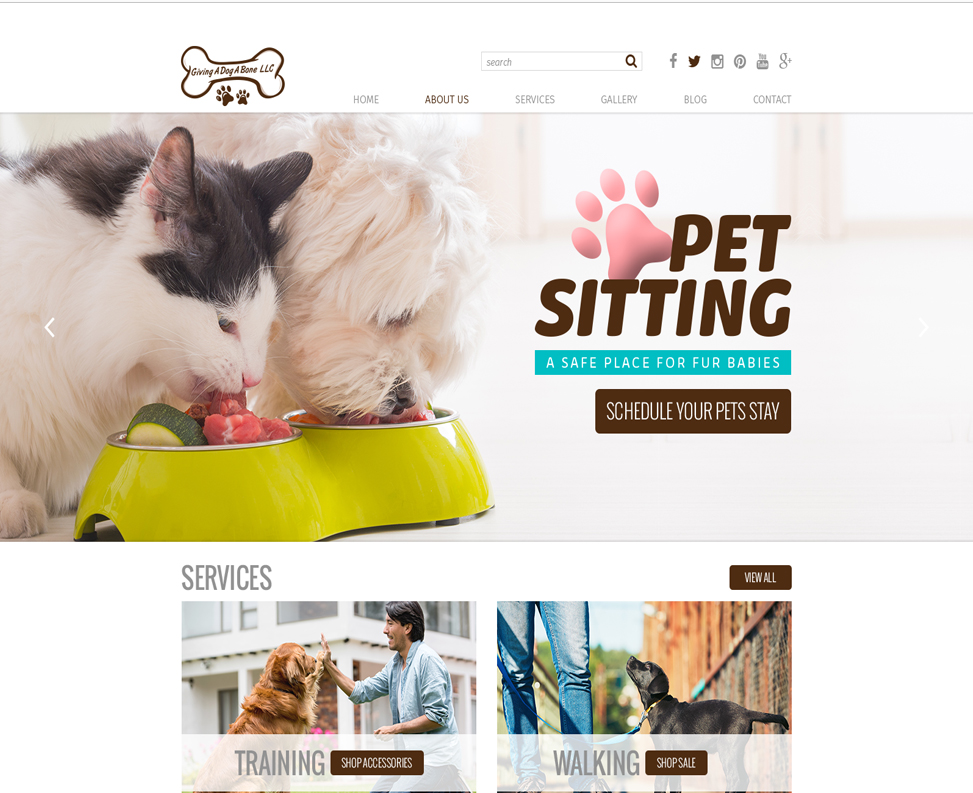This screenshot of a website for "Give a Dog a Bone, LLC" presents a visually appealing and well-organized layout. In the upper left corner, the company's name is displayed alongside its business logo—an intricately designed vector graphic featuring a bone inscribed with the name. Accompanying the logo are two paw prints, adding a playful touch.

To the right of the logo, there's a search box labeled "search," with a magnifying glass icon to its right, making it easy for users to find specific content on the site. Adjacent to the search box are several social media icons: an 'F' for Facebook, a bird symbol for Twitter, a camera for Instagram, a 'P' for Pinterest, a YouTube play button, and a Google Plus icon.

Beneath this header, the main menu offers navigation options including: Home, About Us, Services, Gallery, Blog, and Contact.

The hero image, located just below the menu, features a heartwarming scene of a dog and a cat eating from a food bowl filled with vegetables and fruits. To the right, a banner reads "Pet Sitting: A Safe Place for Babies. Schedule Your Pet Stay," encouraging visitors to consider their pet-sitting services.

The services section includes two columns and a "View All" button in the upper right corner. The first card highlights "Training," with an image of a dog high-fiving a man. The second card, "Shop Accessories," shows a pair of blue jeans standing next to a black dog looking up at them with anticipation, beside the caption "Walking: Shop Sale." The overall design exudes a friendly and professional vibe, perfectly suited for pet owners seeking quality services.